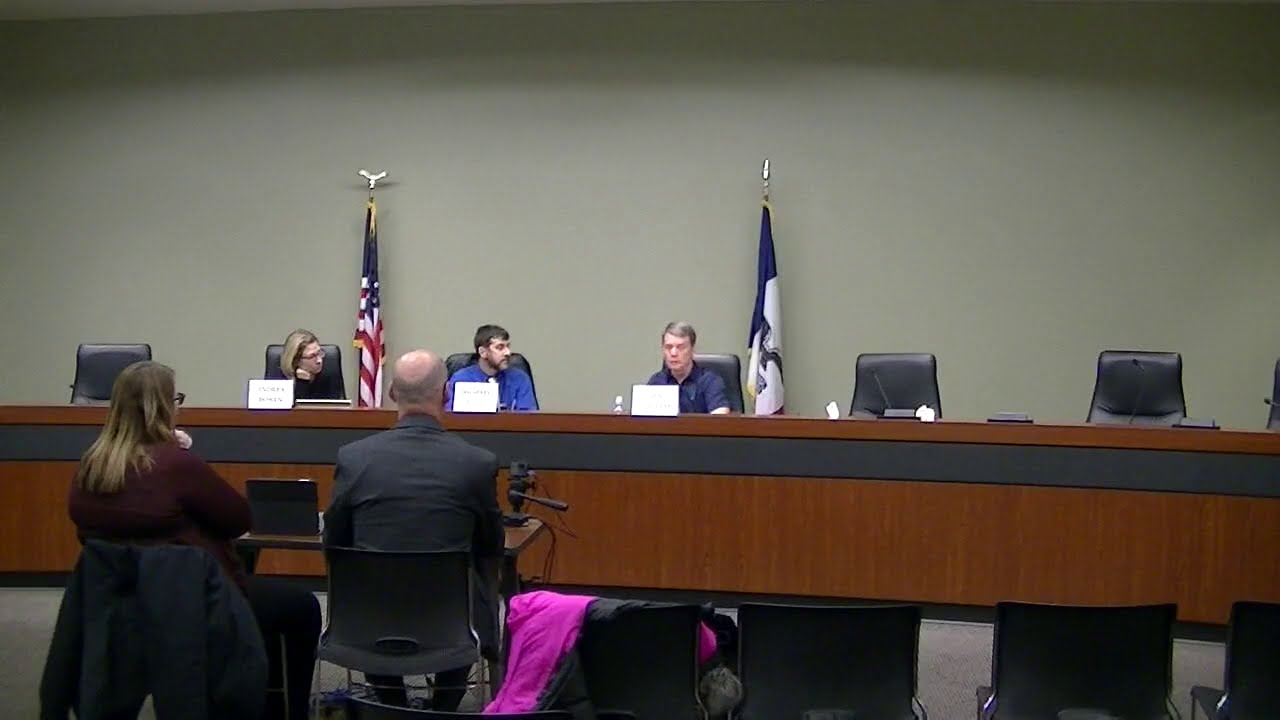In this image, there appears to be a formal city council meeting or a town hall session with a strong air of professionalism. The main focus is a long, wooden podium with a black border on top, behind which three individuals are seated. Toward the left, an older woman with blonde hair and glasses is leaning on her arm, the middle seat is occupied by a man in his 30s or 40s with dark hair, a beard, and a blue button-up shirt, and to the right, an older white man in a collared shirt. Each individual has a white placard in front of them, presumably displaying their names. 

In the background, there is an American flag and a blue and white state flag whose specific state affiliation is unclear. In the foreground, two individuals are seated facing the council; one is a man in a suit with balding hair, and the other is a woman with light brown hair and glasses. Her dark-colored coat hangs off her chair. There are also several empty seats on both sides, indicating that not all positions are occupied. The participants are dressed in business attire, which emphasizes the importance and formal nature of the meeting.